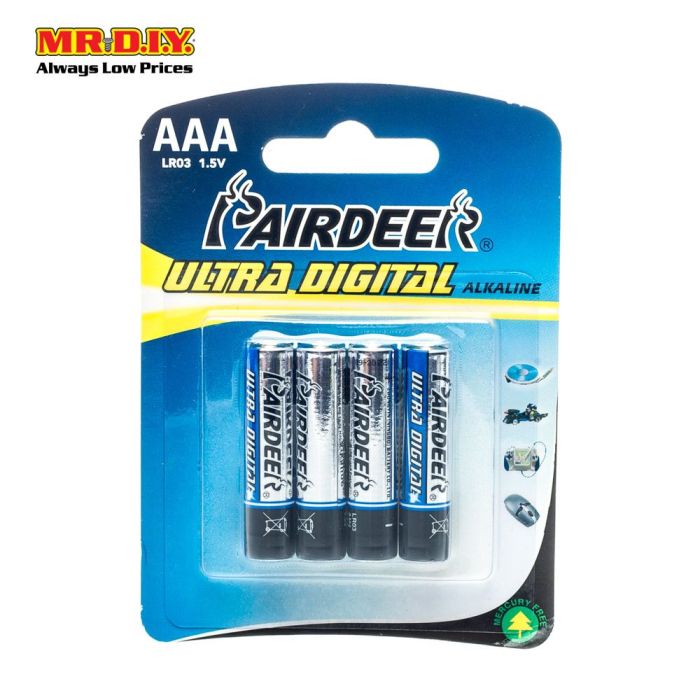The advertisement appears on a web page and prominently features the branding "Mr. DIY" at the top, with the name highlighted in red capital letters and outlined in yellow for maximum visibility. Below this, a tagline in smaller print reads, "Always Low Prices," suggesting that Mr. DIY might be a retail store or an online shop renowned for affordable products.

The main focus of the ad is a package of AirDeer Ultra-Digital Alkaline Batteries, specifically AAA size with a voltage of 1.5V. The packaging is of the standard blister pack variety, with a cardboard backing and plastic bubble sealing the four batteries inside, all oriented with the positive ends facing downward and the negative ends upward.

Alongside the battery pack, there are four smaller images presumably showing compatible devices to highlight the batteries' versatility. These images include a disk drive, a computer mouse, and two other items that appear to be toys, indicating that the AirDeer batteries are suitable for a range of electronic devices. 

Overall, the ad aims to convey the reliability and wide usability of the AirDeer AAA batteries available at Mr. DIY.